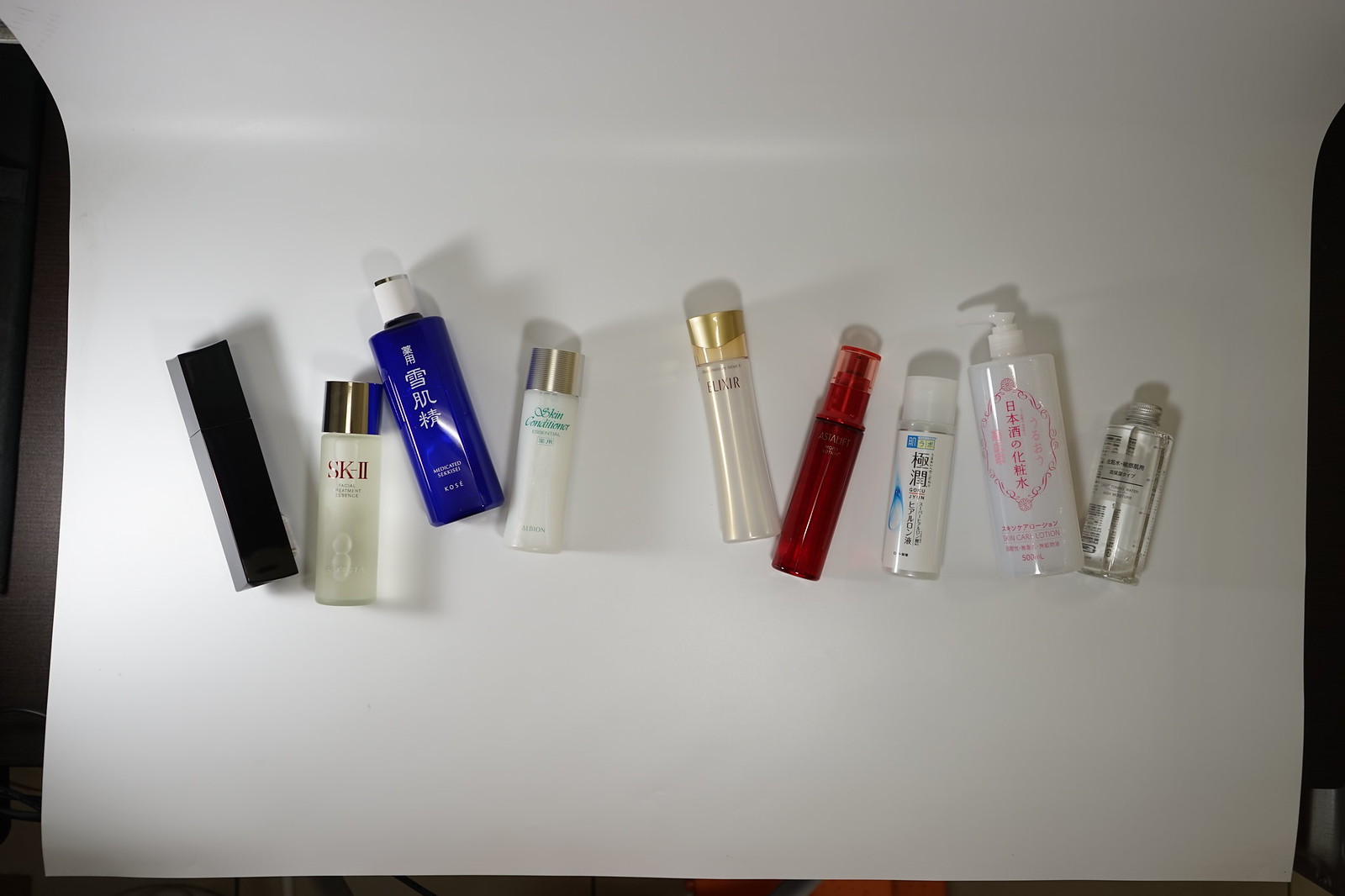This photograph showcases an array of personal care products meticulously arranged on a pristine white surface. Prominently, the collection begins with a sleek, skinny black item, immediately drawing the eye. Adjacent to it is a distinct white bottle adorned with reddish lettering and topped with a silver lid, exuding a sense of elegance. A striking blue bottle with contrasting white font and a matching white cap follows, adding a pop of color to the ensemble. Complementing these is another white bottle, distinguished by its silver lid and embellished with subtle green lettering.

Among the lineup, a clear bottle capped with an opulent gold lid stands out, while a vibrant red bottle with a coordinated red lid introduces a bold splash of color. The composition continues with a tri-colored white, black, and blue bottle, finished with a clear lid, adding a dynamic visual element. A transparent bottle bearing pink font and capped with a white lid provides a softer contrast, alongside another clear bottle with an understated silvery lid, enhancing the diversity of the collection.

The pristine white surface beneath these products not only highlights their varied designs but also casts distinct, crisp shadows, enhancing the three-dimensionality of the scene. At the periphery, hints of various colors, including some subtle blacks and a touch of orange, frame the central display. The surface itself reflects light gently, imparting a glossy, polished look that adds to the overall aesthetic appeal of the photograph.